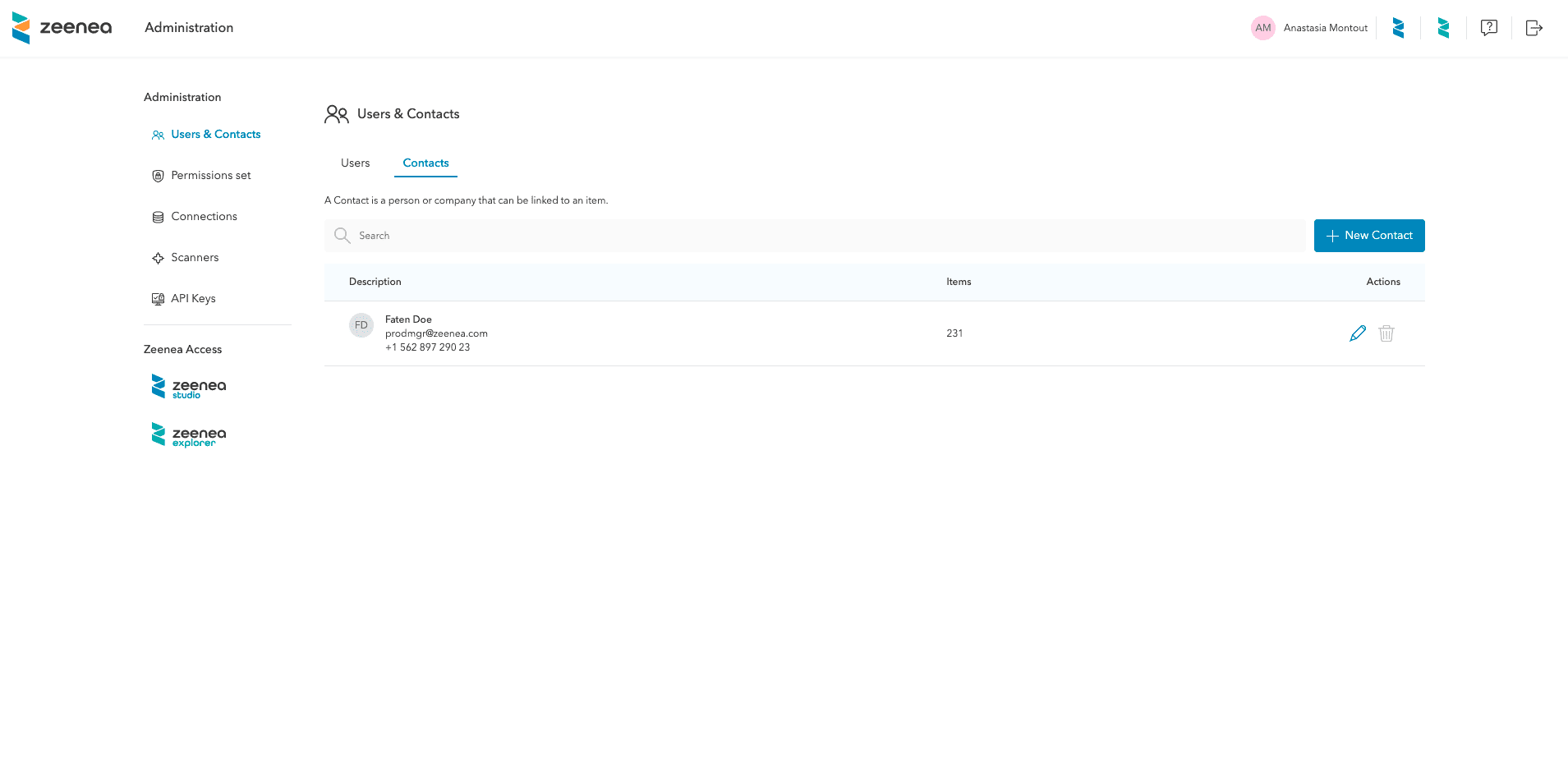The image features a complex composition of symbols, colors, and text. At the center-left, there is a prominent symbol colored in blue and yellow, accompanied by two partially indistinguishable words. To the right, a pink circle contains letters and is adjacent to a blue squiggle and a green squiggle. Below these elements, there is a box with an unclear content and a right-pointing arrow.

On the left-hand side, there is a word in black text, below which is a blue symbol followed by several words in black. Another symbol is located next to a word in black, along with yet another symbol leading to more black text. The blue squiggle appears again, flanked by words in black and blue.

The bottom section of the image displays symbols representing two people with corresponding text nearby. A word in black is located to the left of a blue-underlined word, followed by additional black text. Adjacent to this is a gray rectangle and a blue rectangle containing text. Further along, a light blue rectangle with text and a gray circle featuring unreadable content are present.

Finally, towards the middle, there is an undefined element and a blue pencil symbol, accompanied by a very light gray symbol towards the bottom of the image. The overall layout is intricate, featuring a mix of colors, shapes, and text elements, each contributing to the depth and complexity of the visual presentation.